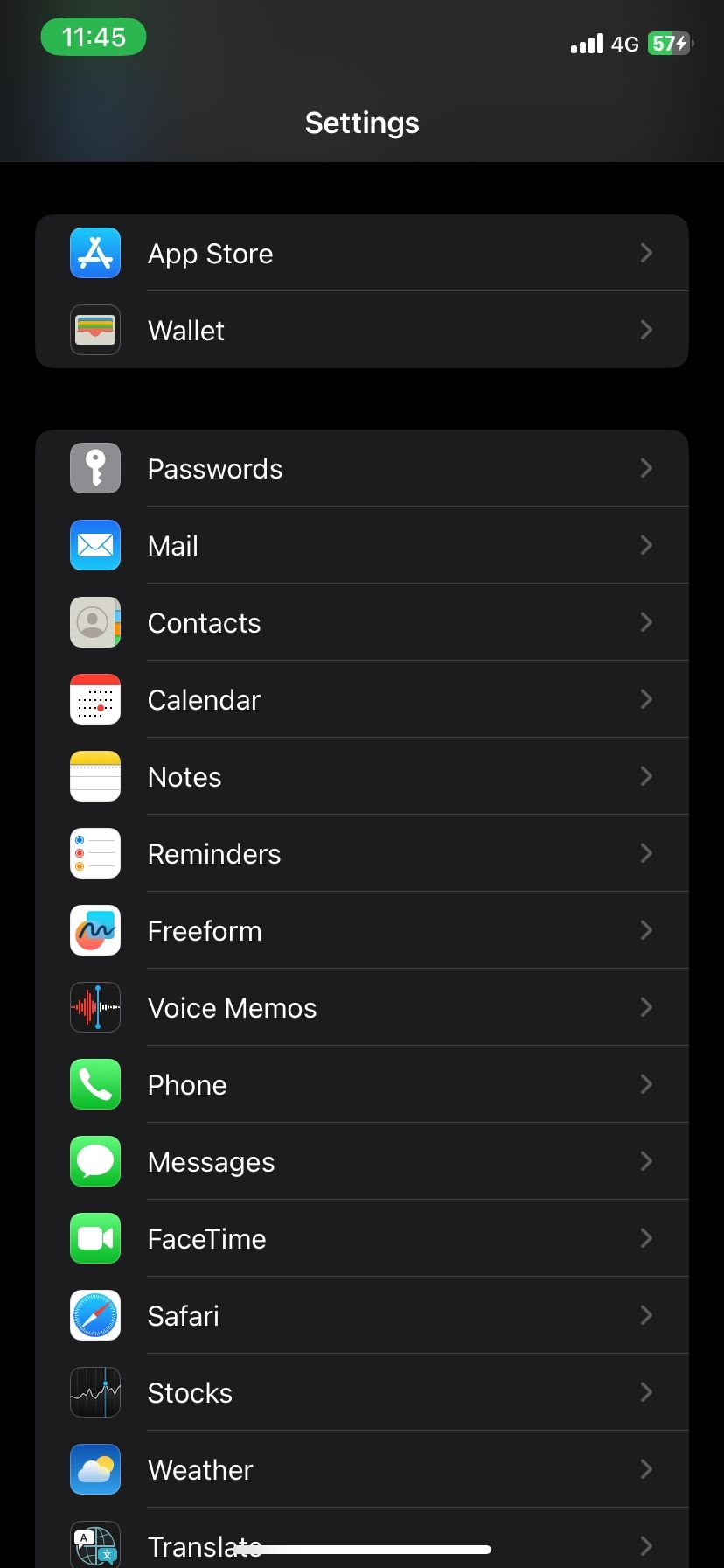The image depicts the screen of a smartphone against a black background. In the top left corner, there is a green oval containing the time "11:45" in white text. On the top right side, the screen shows four bars indicating strong cellular reception, a "4G" label in white, and a battery icon. The battery shows 57% charge, with the percentage displayed in green within the battery icon. The remaining part of the battery icon is gray and includes a lightning bolt, indicating that the phone is currently charging.

Directly below the status bar, there is a central section displaying two applications in white text: "Settings" and "App Store," each within a dark gray rectangle. The titles are separated by a thin white line.

Further down, there is a series of white text labels representing various app categories and features, each separated by a thin gray line. The labels read, in order: "Passwords," "Mail," "Contacts," "Calendar," "Notes," "Reminders," "Phone," "Voice Memos," "Messages," "FaceTime," "Safari," "Stocks," and "Weather." Each label has a line beneath it, maintaining the consistent gray divider between the categories.